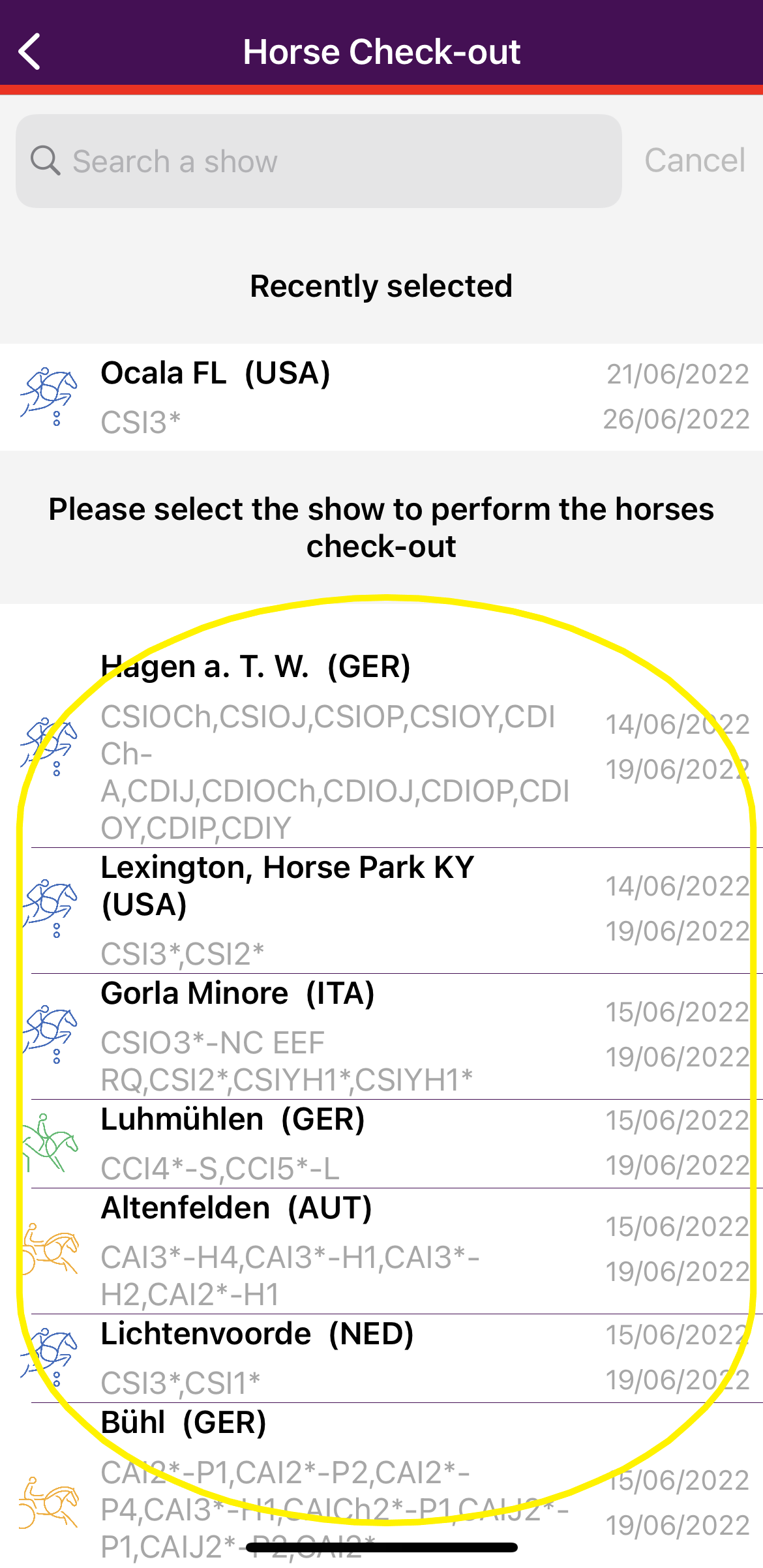The website interface displays a section titled "Horse Checkout," characterized by a dark purple bar at the top. On the left side of this bar, there is a back arrow icon underlined by a thin red bar. Below this, a gray section provides a search function labeled "Search a Show" with a "Cancel" option beside it. 

The main content area lists "Recently Selected" items, featuring an entry for Ocala, Florida, USA, accompanied by a 2022 date and a designation of "CS 13." The prompt instructs users to "please select the show to perform the horse's checkout."

A noticeable yellow circle highlights several horse names along with their respective events and locations, detailed as follows:
- Hagen ATW, Lexington Horse Park, Kentucky
- Gore Gorilla, Menor, Italy
- Alton Felden, Australia
- Lichten Rorty, Netherlands
- Buell, Germany

Each horse's entry is visually represented with icons in various colors like yellow, green, and blue, displayed on the left-hand side, while the dates they were selected are shown on the right-hand side.